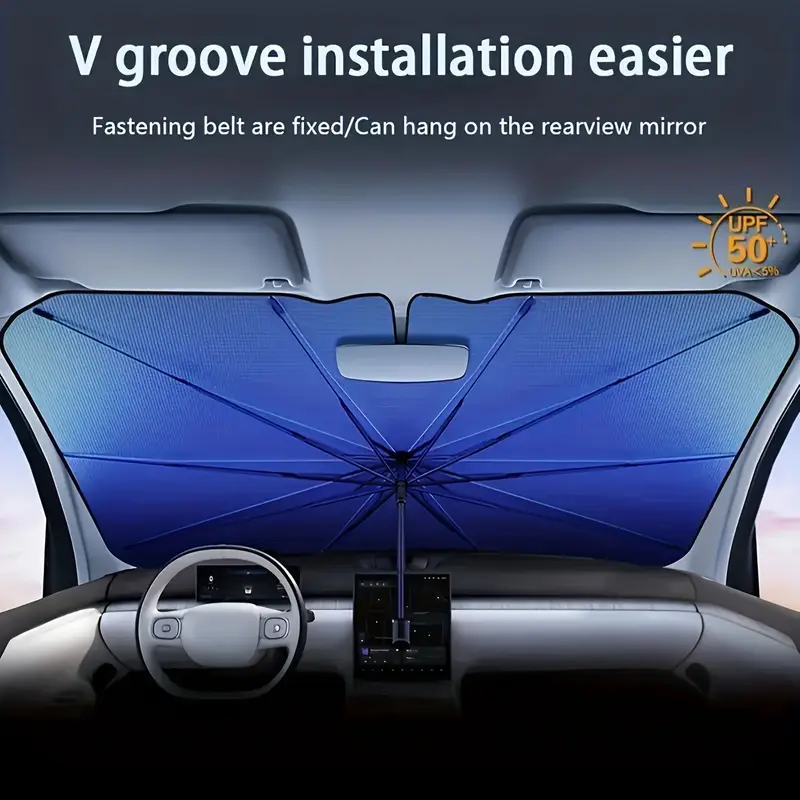This advertisement features the interior of a modern car with a blue sunshade covering the entire windshield. The sunshade, which unravels in an umbrella-like fashion and wraps around the rearview mirror, is prominently marked with a UPF 50+ logo in yellow, indicating high sun protection. The top of the ad includes text that reads, "V-groove installation easier. Fastening belt are fixed / can hang on the rearview mirror," highlighting its user-friendly setup. The sunshade also showcases a distinctive spiky design, emphasizing its unique structure and functionality.